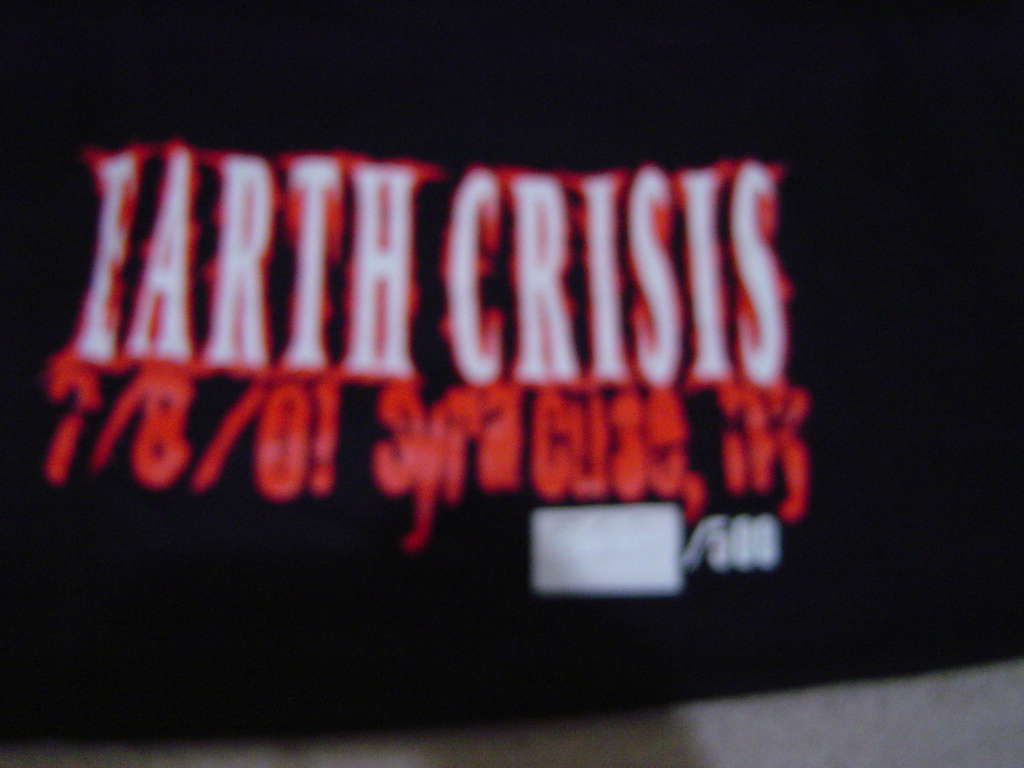The image features a black textile, possibly a banner or t-shirt, suspended against a concrete floor or wall. The text "Earth Crisis" is prominently displayed in bold white letters, outlined in red. Below it, "7801 Syracuse, New York" is written in red. A white, opaque rectangle obstructs a portion of the text, which seems to indicate the item's limited edition number out of 500. The photograph is poorly taken, either zoomed out or unclear, with the edges of the material cut off, making it difficult to determine the exact nature of the item and its surroundings.